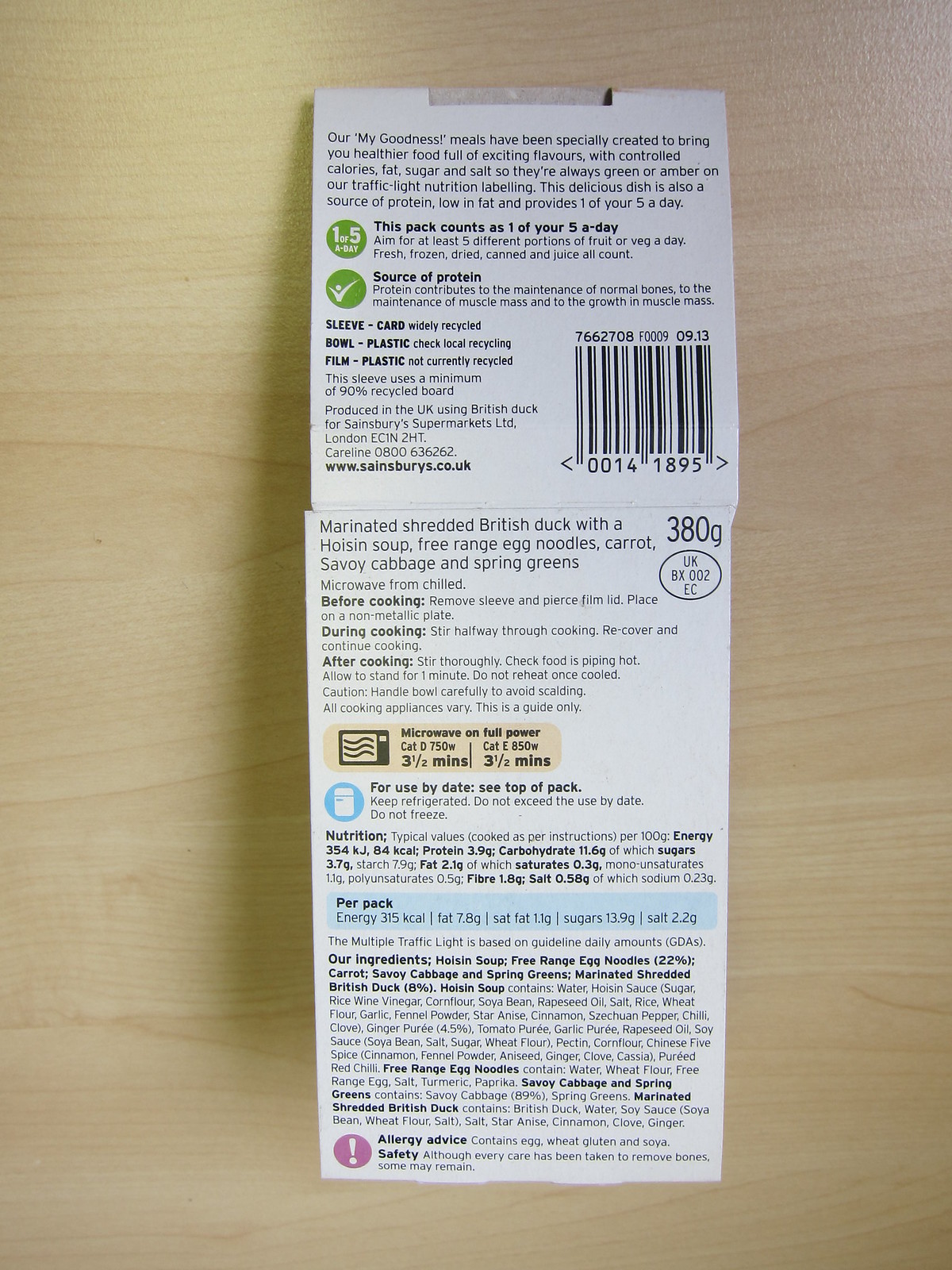A nutrition label is displayed on a wooden table. The label itself is white with black lettering and features some green logos. It reads as follows: "Our My Goodness Meals have been specially created to bring you healthier food full of exciting flavors with controlled calories, fat, sugar, and salt. They are always green or amber on our traffic light nutrition labeling. This delicious dish is also a source of protein, low in fat, and provides one of your five a day. Aim for at least five different portions of fruits or vegetables daily—fresh, frozen, dried, canned, and juices all count." The label is the focal point, with the specific product it belongs to remaining unidentified.